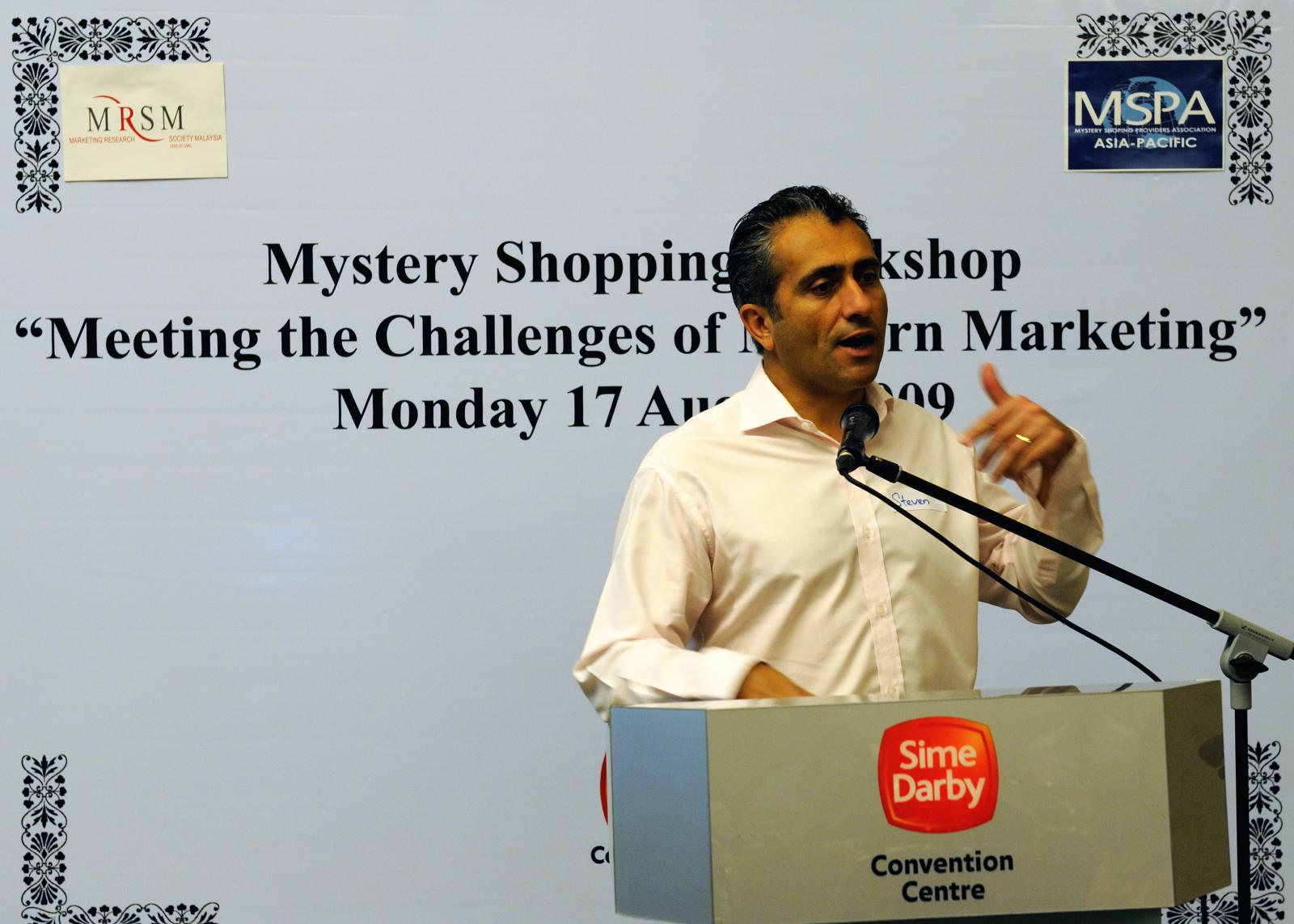The image captures a man with dark skin and dark features, including black hair and dark eyebrows, speaking into a microphone while standing at a gray and blue podium. He is partially obstructed by the podium, and is wearing a light-colored, cream dress shirt with a possible insignia on the left chest area. Notably, he has a wedding band on his left ring finger, which is raised as he gestures while speaking. The backdrop consists of a light gray or blue wall which displays partially obscured text: "Mystery Shopping Workshop, Meeting the Challenges of Marketing," followed by "Monday, 17th August," with a potential year of 2009, though this part is obscured by the man. The podium bears the logo of "Sime Darby" in white lettering on an orange background, along with the words "Convention Center" in black text. The background also features two additional logos reading "MRSN" and "NSPA." The man’s posture, with his mouth slightly open, suggests he is engaging in a speech or answering a question during the event.